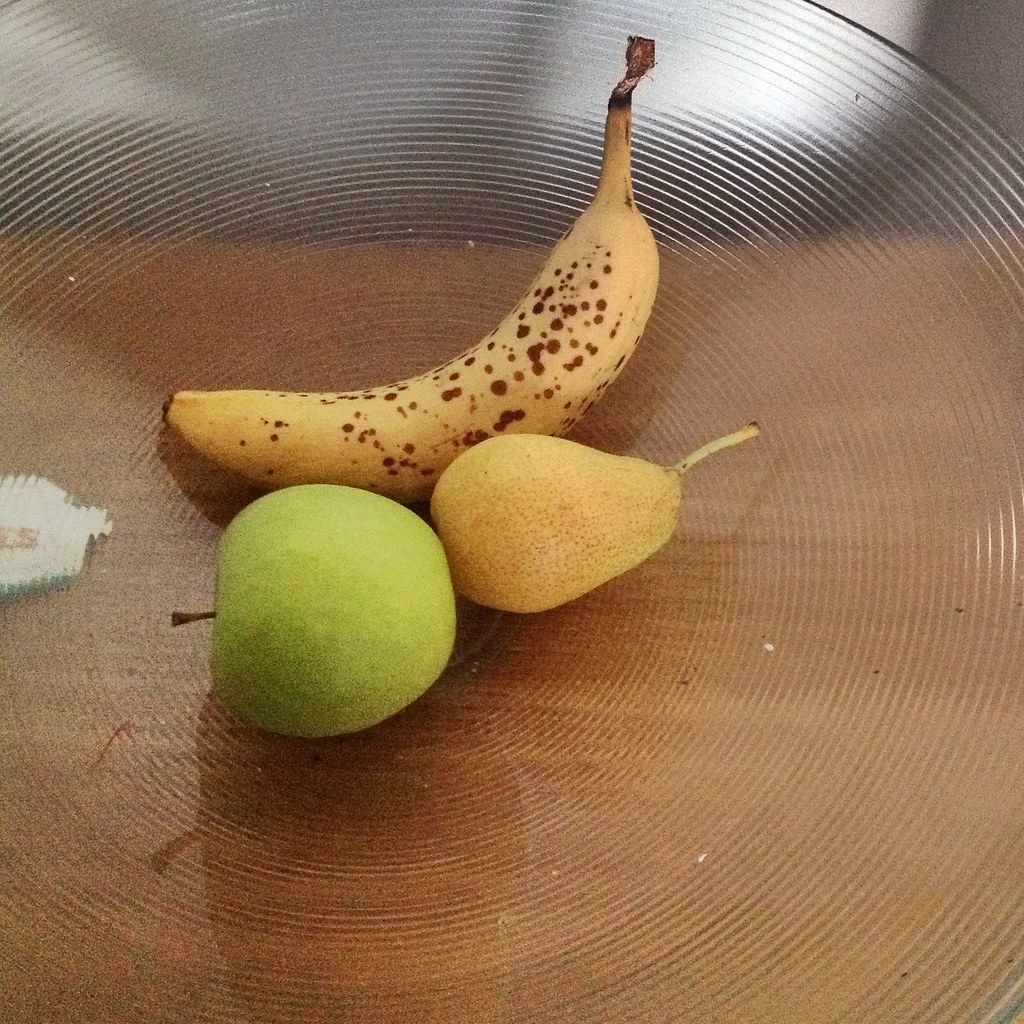A clear bowl with distinctive lines is the central focus, positioned on a wooden table. The bowl is illuminated from the right side, casting a soft gray light that enhances the transparency and the intricate line patterns of the bowl. Through the clear glass, the texture of the wooden surface beneath is distinctly visible. To the left of the bowl, an indeterminate patch featuring white, gray, and some red lettering can be seen, partially obscured by the bowl's design. Inside the bowl, there is a small, yellow banana speckled with brown spots, standing upright with its stem on the right and the brown-tipped end on the left. Accompanying the banana is a green apple lying on its side, with its stem oriented to the left. Additionally, a small, yellowish pear with a rightward-pointing stem completes the composition within the bowl. The fruits, displaying varying degrees of ripeness, add a vibrant contrast to the clear, structured setting of the bowl.